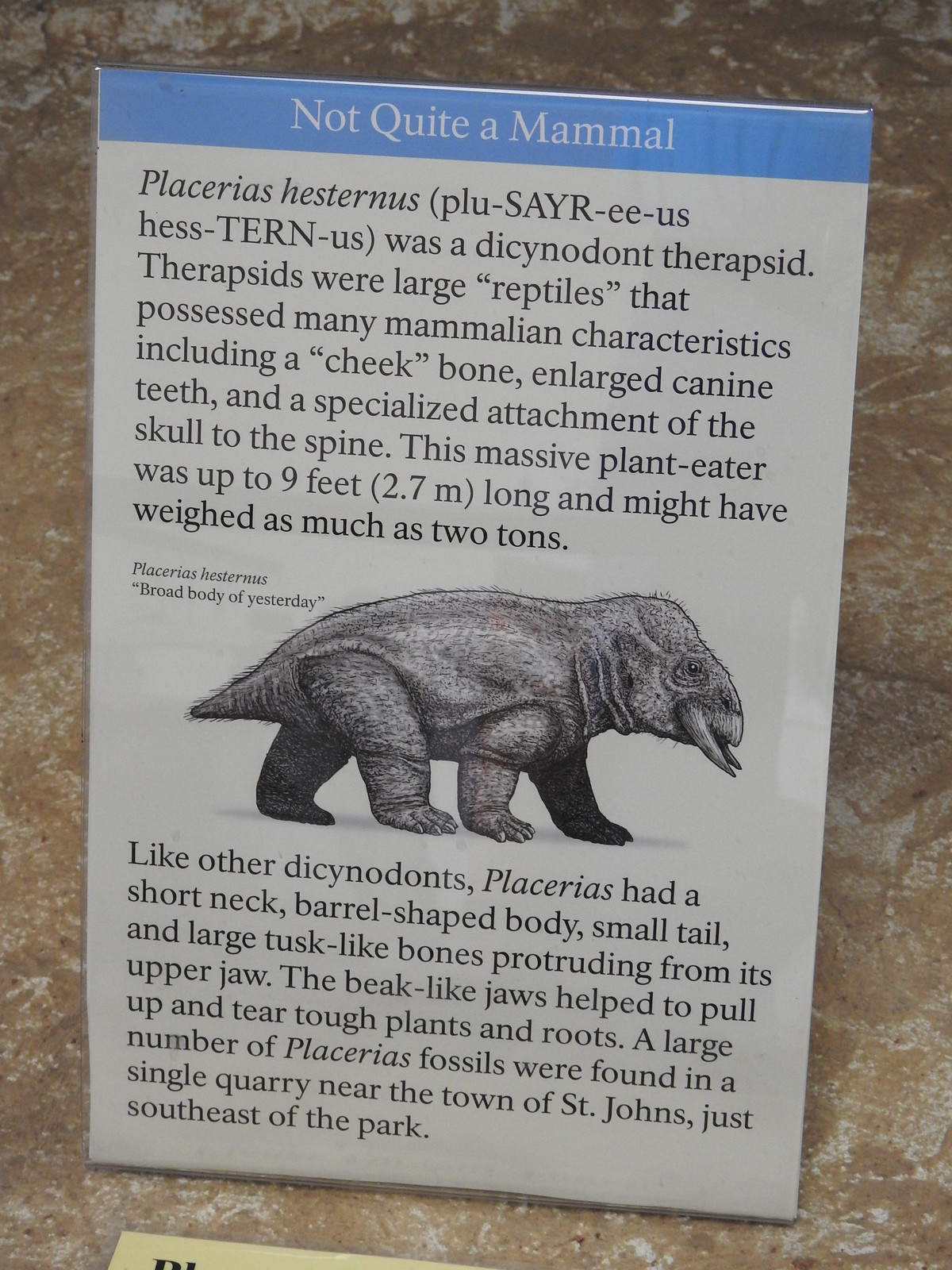The image appears to be of an informational display, likely from a museum and designed for children due to its simple, clear language. The display has a blue top border with white lettering that reads "Not Quite a Mammal." The main focus is a black and white drawing of a prehistoric reptilian creature named Placerias hesternus, which visually resembles a cross between an elephant and a rhinoceros. The text provides detailed information about the creature, noting that it was a plant eater with enlarged canine teeth, measured nine feet in length, and weighed up to two tons. The fossils of Placerias hesternus were discovered in a single quarry near the town of St. Johns, indicating its historical habitat.